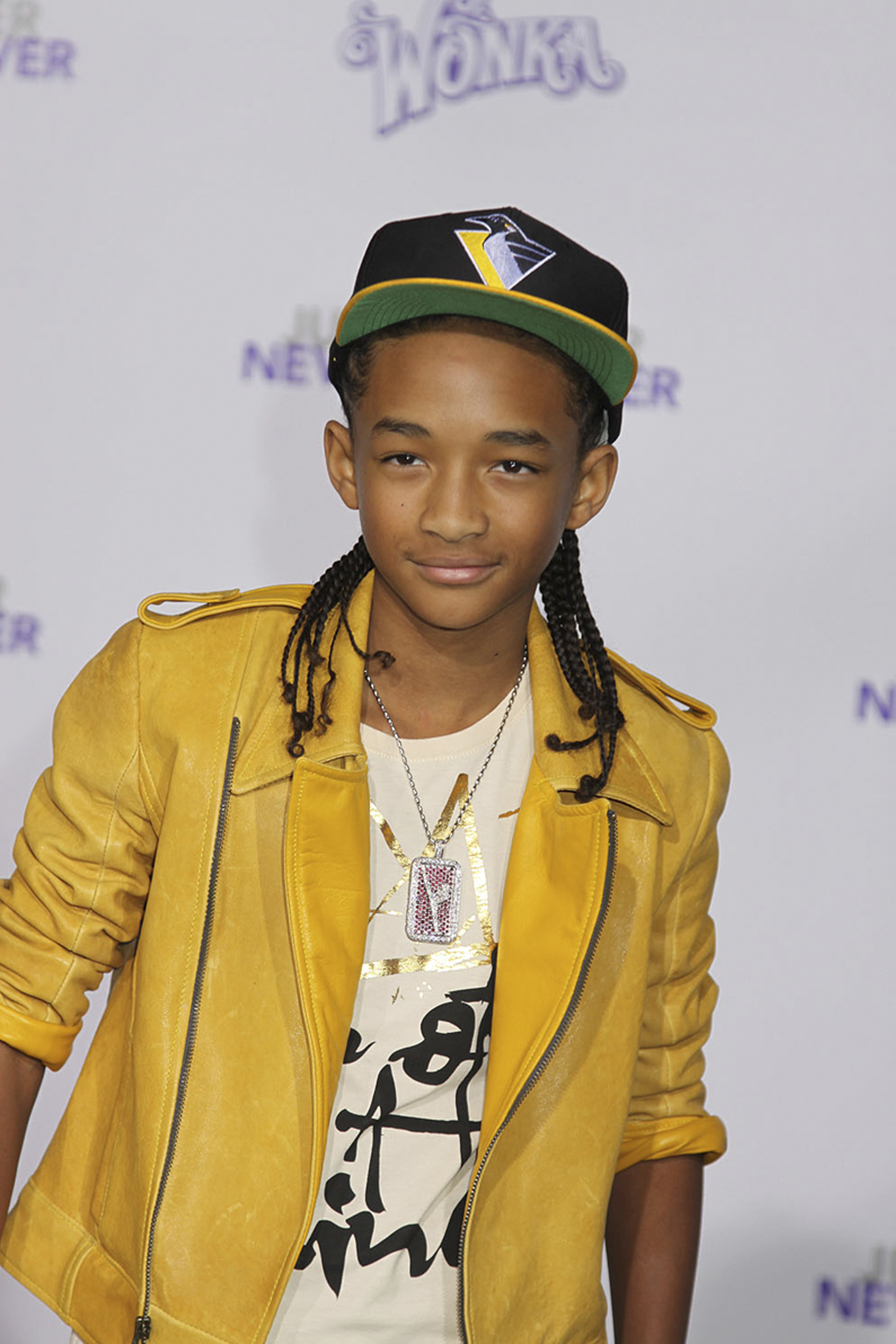In this image, a young Jaden Smith, the son of Will Smith and Jada Pinkett Smith, is seen leaning slightly to one side with a subtle, closed-mouth smile. His darker golden skin and cornrow braids cascading down the back are prominent features. Jaden is wearing a black Pittsburgh Penguins baseball cap, which is slightly oversized, revealing his entire forehead. The hat has green and yellow trim. He is dressed in a yellow leather jacket with long sleeves rolled up to his elbows, over a white t-shirt that features black writing and hints of gold. Around his neck, Jaden sports a necklace with a distinctive pink and white diamond-plated pendant. Behind him, the blurry, white background prominently displays the words 'Willy Wonka,' suggesting he might be attending an event related to a movie.